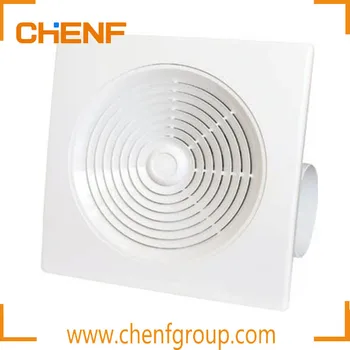The promotional image showcases a white exhaust fan nestled within a white plastic casing, positioned centrally against a square background. The fan features a circular vent in the middle designed for airflow, with a white pipe protruding from the back. Enhanced with four unconnected orange right-angle markers in each corner, the image is bordered, providing a striking visual frame. In the upper left corner, the brand name "CHENF" is prominently displayed in a bold orange blocky font, with a distinct blue box forming the upper right segment of the letter "H." At the bottom center of the image, the manufacturer's website, "www.chenfgroup.com," is presented in a slim orange font. The meticulous layout and branding elements, coupled with the clear depiction of the exhaust fan, suggest that this is an advertisement image aimed at highlighting the product's design and functionality.